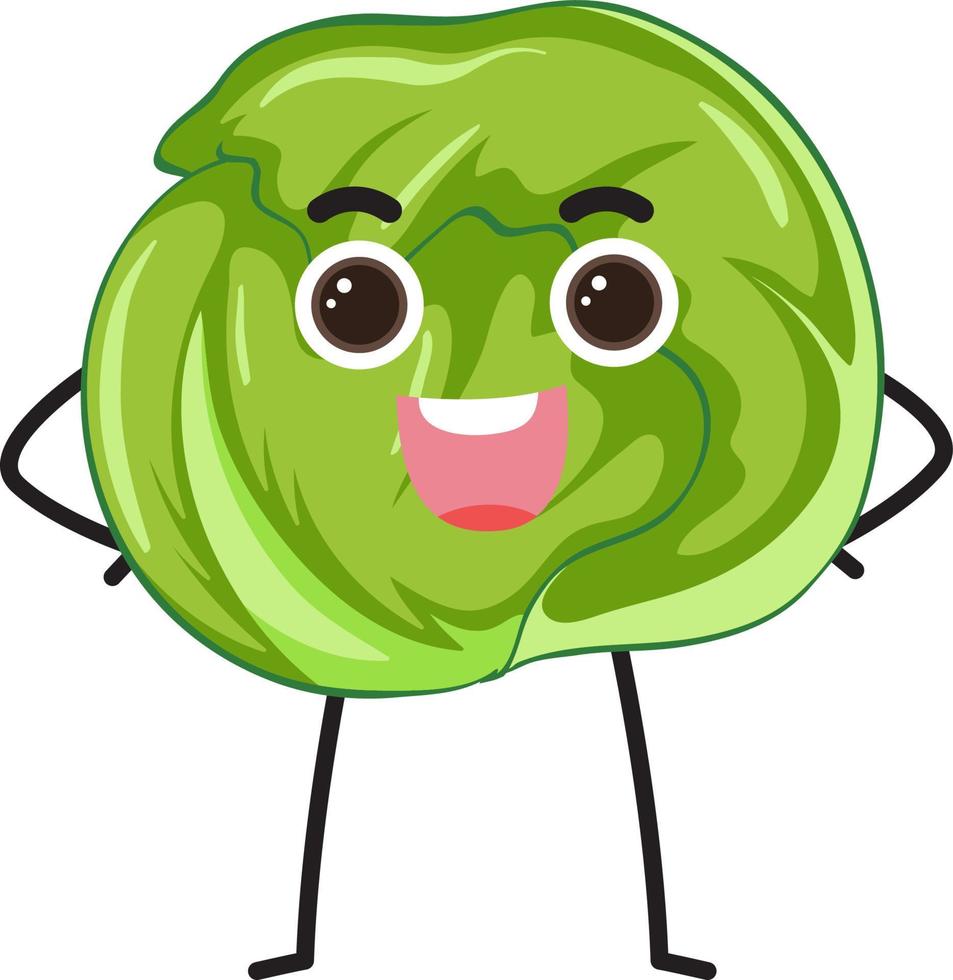This image is a detailed clip art illustration of an anthropomorphic vegetable, resembling a head of lettuce or cabbage. The character is primarily light green, with shading in darker greens and lighter shades to add depth. Its most striking features are its large, expressive eyes, which have white sclera with dark brown irises, and black pupils. The eyes are positioned directly forward beneath prominent eyebrows. The mouth is an open U-shape, revealing a single white tooth and a pink tongue at the bottom, with the inside of the mouth also rendered in pink.

The character has thin, black line-drawn arms and legs, simple stick figure-like limbs. The arms are bent so that what serves as the hands are positioned on the lower half of its body, suggesting an assertive yet joyful stance. The overall impression is one of happiness and cheerfulness. The head or main body of the character has a lumpy, leafy appearance, almost like hair, which emphasizes its plant-like nature. It exudes a playful and friendly demeanor.